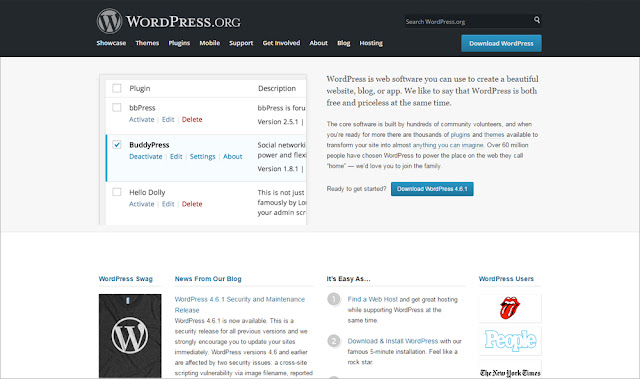The caption provided has been revised and detailed for clarity and completeness:

"This image is a screenshot of the homepage of WordPress.org. At the top, there is a black banner featuring white text that reads 'WordPress.org,' and a navigation menu with options such as 'Showcase,' 'Themes,' 'Plugins,' 'Mobile,' 'Support,' 'Get Involved,' 'About,' 'Blog,' and 'Hosting.' A search box is also available for site-specific searches. Adjacent to the search box, there is a prominent blue button labeled 'Download WordPress.'

Below the banner, the layout includes an image on the left and text on the right. The image appears to display a selection of plugins, including bbPress, BuddyPress, and Hello Dolly, suggesting these are available plugins for WordPress. The accompanying text reads: 'WordPress is web software you can use to create beautiful websites, blogs, or apps. We like to say that WordPress is both free and priceless at the same time.'

Beneath this section, more text and a few links are present, albeit blurry. Another blue button labeled 'Ready to get started? Download WordPress' is visible, although the version number is indistinct.

Further down, there is a small image of a black rectangle with a stylized 'W' representing WordPress next to the phrase 'WordPress Blog.' To the right, there's text inviting users to 'Read the news from our blog.' Following this, the layout showcases different sections with links that provide information on how to 'Find a Web Host' and 'Download and Install WordPress.'

On the far right side of the row, there's an iconic image of the Rolling Stones' lips and tongue logo, signifying that the Rolling Stone magazine uses WordPress. Additional mentions indicate that prominent entities like 'People' and 'The New York Times' also utilize WordPress."